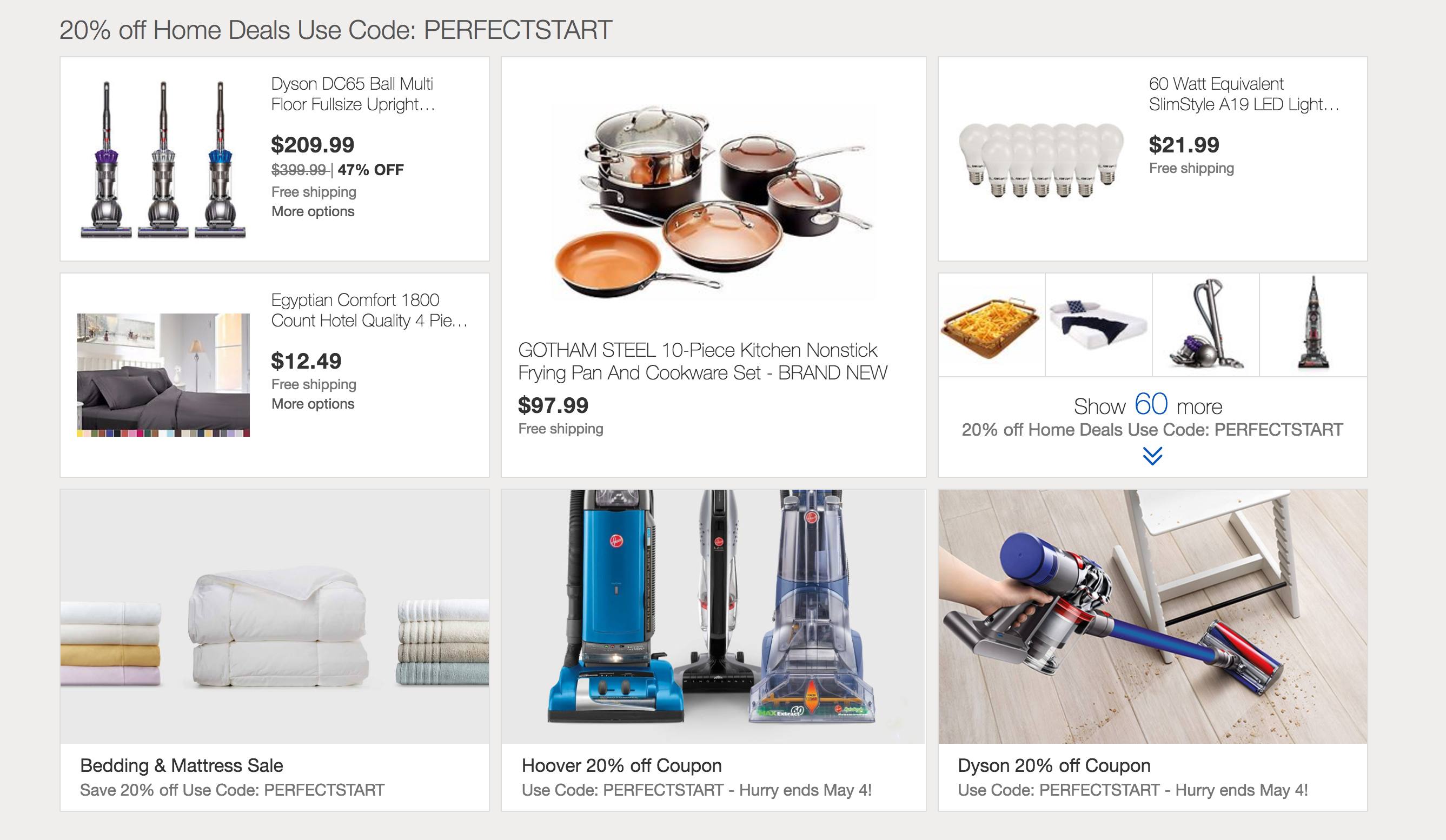On this page, 20% of home deals can be availed by using the code PERFECTSTATS. The listings include:

1. **Dyson BC65 Ball Multi-Floor Full-Size Upright Vacuum** - Originally priced at $399.99, now available for $209.99, offering a significant discount of 47.6%. This deal includes free shipping.
2. **Egyptian Comfort 1800 Count Hotel Quality 4-Piece Bedspread** - Priced at a mere $12.49, this luxurious bedspread comes with free shipping.
3. **Gotham Steel 10-Piece Kitchen Non-Stick Frying Pan and Cookware Set** - A brand-new set priced at $97.99.
4. **60-Watt Equivalent Slim Style A19 LED Light** - Available for $21.99.
5. **Discount Coupons**:
   - **Dyson 20% Off Coupon**: Use code PERFECTSTATS. Hurry, this offer ends on May 4th.
   - **Hoover 20% Off Coupon**: Use code PERFECTSTATS.
   - **Bed in a Mattress Sale**: Save 20% by using the code PERFECTSTATS.

Be sure to take advantage of these deals by using the provided discount code PERFECTSTATS before they expire.